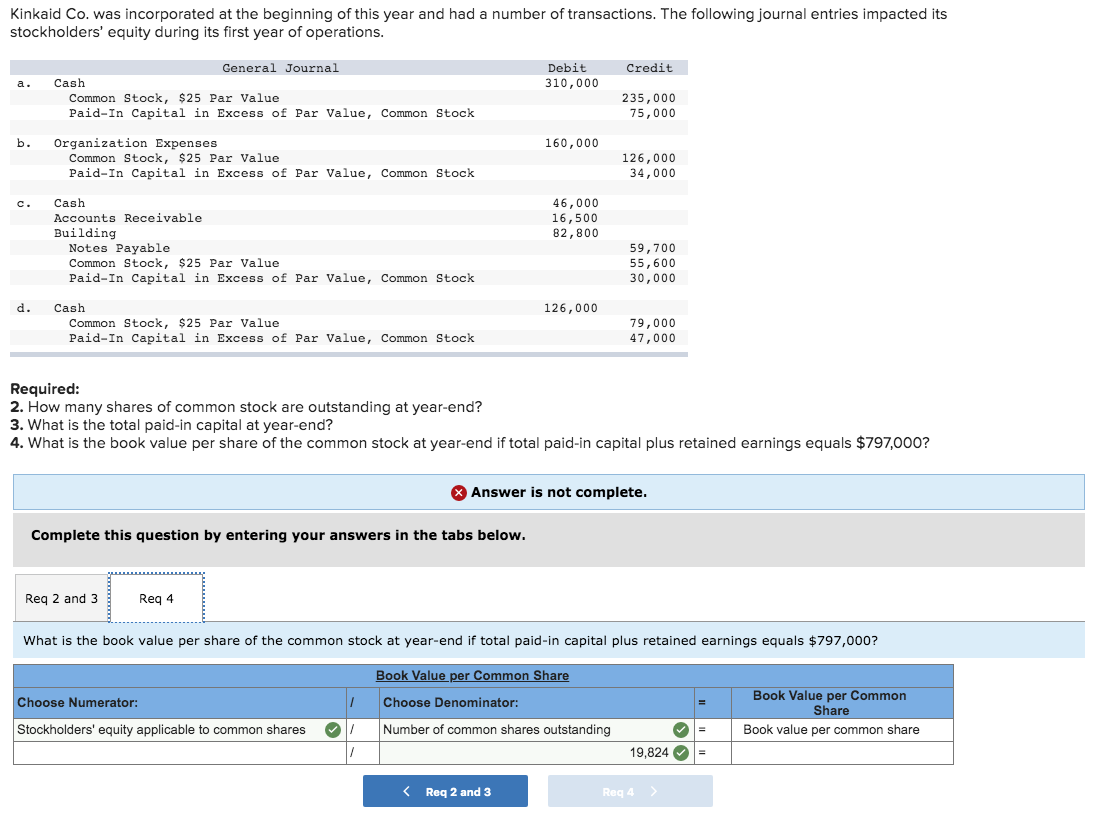The image displays a screenshot of a detailed journal entry, illustrating various transactions related to stakeholder equity. At the top, under the heading "General Journal," several debits and credits are listed. 

1. **Transaction A**:
   - **Accounts**: Cash, Common Stock ($25 par value), Paid-in Capital in Excess of Par Value - Common Stock
   - **Amounts**: 
       - Debit: $310,000 (Cash)
       - Credit: $235,000 (Common Stock)
       - Credit: $75,000 (Paid-in Capital)

2. **Transaction B**:
   - **Accounts**: Organizational Expenses
   - **Amounts**:
       - Debit: $160,000
       - Credit: $126,000
       - Credit: $34,000

3. **Transaction C**:
   - **Accounts**: Accounts Receivable, Buildings, Notes Payable
   - **Amounts**:
       - Debit: $46,000 (Accounts Receivable)
       - Debit: $16,500 (Buildings)
       - Debit: $82,800 (Notes Payable)
       - Credit: $59,700
       - Credit: $55,600
       - Credit: $30,000

4. **Transaction D**:
   - **Accounts**: Cash, Common Stock
   - **Amounts**:
       - Debit: $126,000 (Cash)
       - Credit: $79,000 (Common Stock)
       - Credit: $47,000 (Additional Capital)

The screenshot also includes a secondary section below the journal entries, where the user can answer related questions or complete the task.